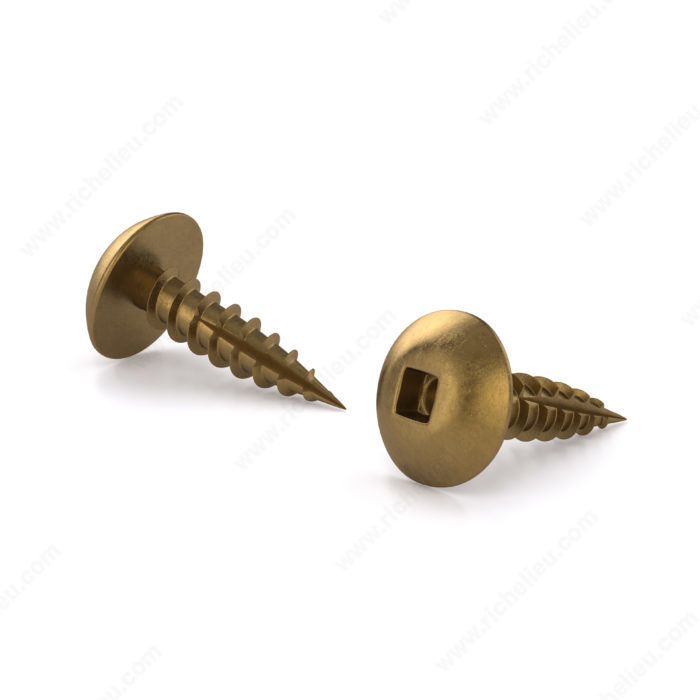The photograph depicts two shiny, bronze-colored screws against a plain white backdrop, with subtle shadows cast beneath them. Both screws are distinctively large in the frame and exhibit prominent spiral ridges along their lengths, tapering to sharp points. The screw positioned on the right is oriented towards the camera, prominently displaying its flat head with a square hole, suggesting the need for a square-headed or Allen wrench screwdriver. The screw on the left is angled slightly away from the camera, revealing more of its spiraled body. The white background is largely unadorned, with a faint and only barely discernible website URL, www.richellen.com, adding a minimalistic touch to the overall simplicity of the image.